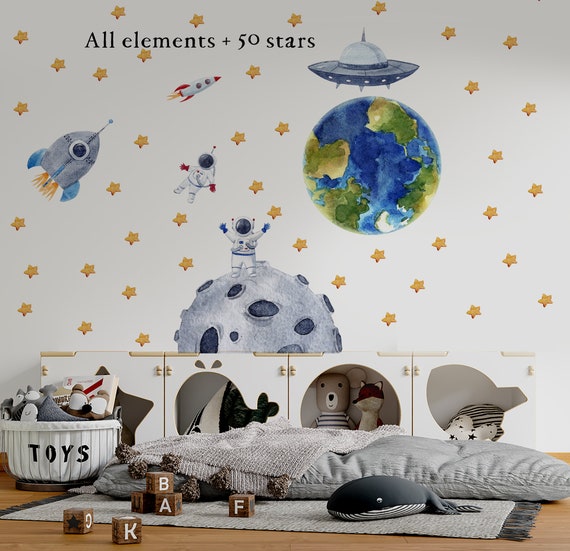This is a detailed color photo of a child's space-themed bedroom. The background features a whimsical wallpaper with a white base adorned with numerous yellow stars, and an inscription at the top in black letters reading "all elements plus 50 stars." Prominently displayed on the wall are several space-themed elements: a blue and green watercolor-like depiction of Earth, a hovering gray alien spaceship, a chunky blue rocket ship and a sleek red and white rocket ship, along with two astronauts—one floating above and another standing on a cratered gray moon. The astronaut on the moon has blue gloves, while the floating one has red gloves.

Below this engaging mural, the room's floor is a mix of hardwood and a gray carpet, which hosts a variety of playful items. There is a dark gray stuffed whale lying on a rug in the center of the room, alongside lettered wooden blocks displaying the letters G, K, B, A, and F. To the left, a white basket labeled "TOYS" in black lettering is filled with an assortment of children's toys. Adjacent to it is a white cabinet with animal-shaped cutouts, housing more plush toys, including a kangaroo and a fox. Additionally, the room contains a large gray pillow and a sleeping bag, adding to the cozy ambiance. The overall scene exudes a sense of adventure and comfort, perfect for a young space enthusiast.